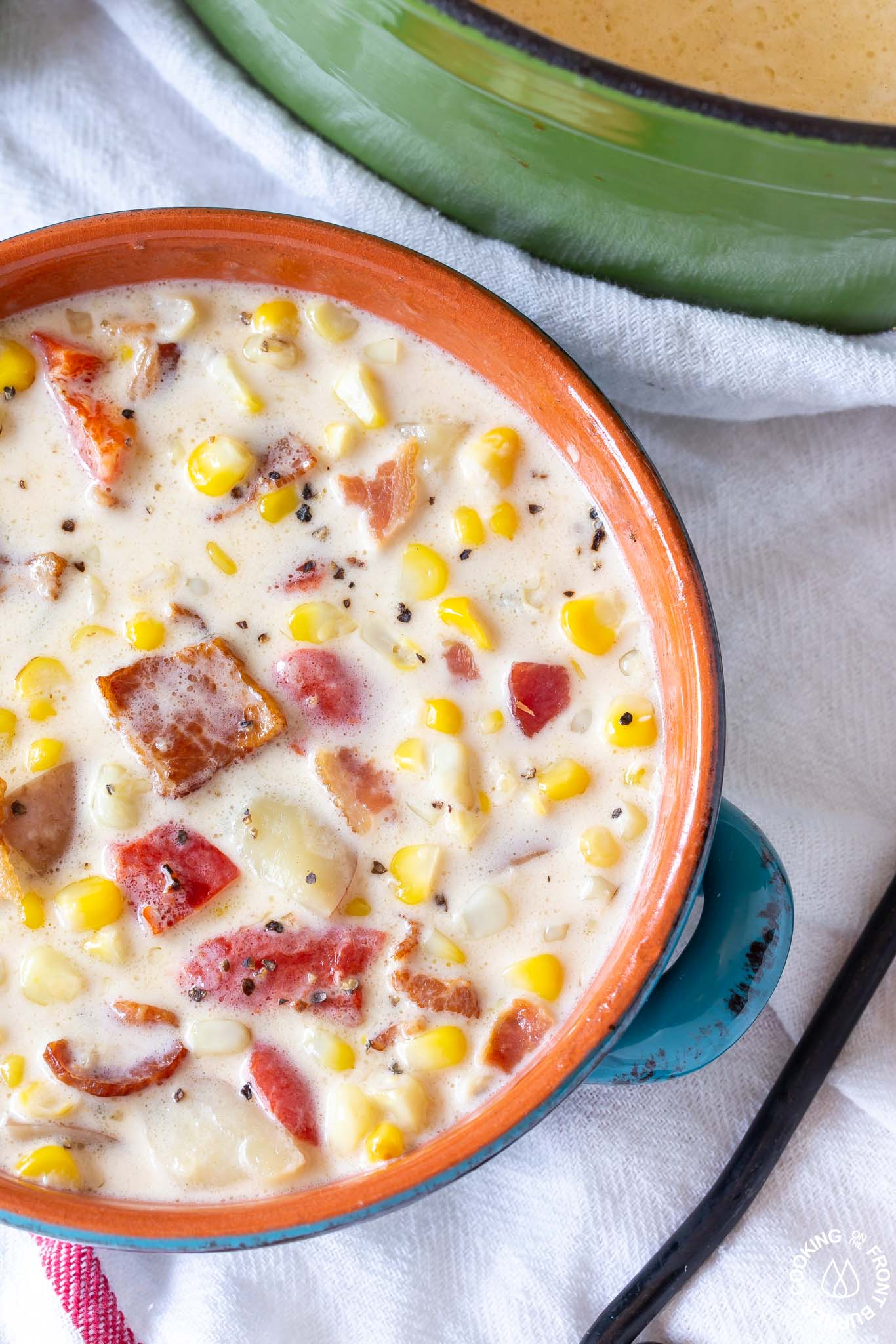The image is a detailed, close-up photograph of a hearty bowl of clam chowder, featuring a thick, semi-frothy, white broth filled with ingredients like sweet corn, diced tomatoes, and what appears to be crispy bacon bits. The chowder is served in a distinctive bowl with an orange interior and a blue exterior, its right handle visible near a black bar that rests on a pristine white cloth. Positioned above and slightly to the right of the bowl is a green container filled with a cheese-colored substance, possibly shredded cheese or a soft cheese dip. The scene is set against a white napkin on a table, suggesting a neatly arranged setting, perhaps for a food blog or social media post. In the bottom right corner, a logo partially obscured by light reads "COOKING FRONT," adding a professional touch to the presentation.